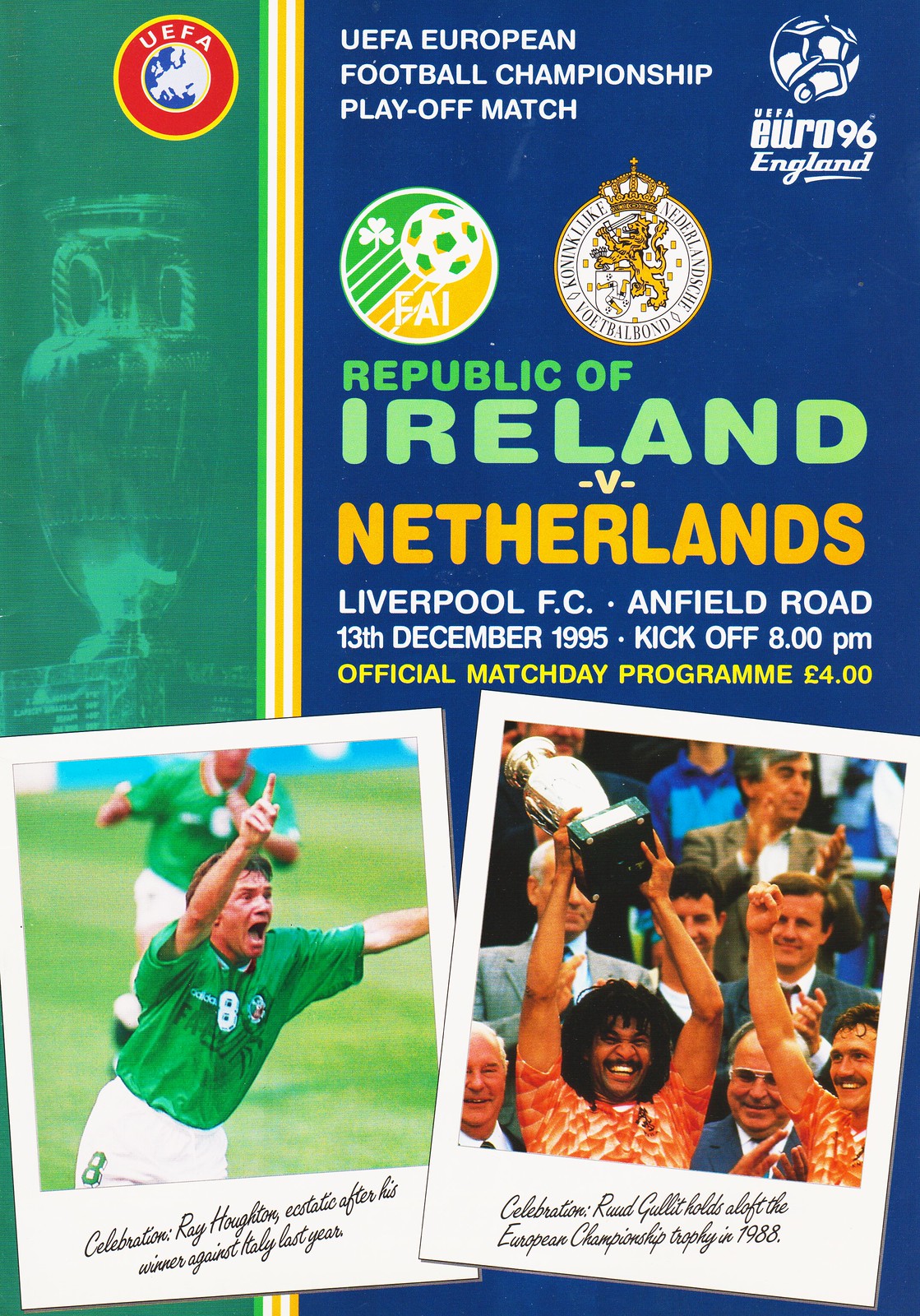The cover of the UEFA European Football Championship Playoff Match program is visually striking and detailed. Dominating the upper left corner is a red and yellow circle with "UEFA" inscribed, while the adjacent text announces the UEFA European Football Championship Playoff Match. The upper right corner features a white soccer ball illustration on a blue background with the text "UEFA Euro 96 England." Below this are two logos: the first is a green, yellow, and white circle with a soccer ball and a four-leaf clover, inscribed with "FAI" representing one of the teams. The second logo, although smaller and difficult to read, is a white circle with a gold line in the center and a crown above a lion's head.

Continuing down, green text names the competing teams: "Republic of Ireland" prominently displayed, followed by "Netherlands" in yellow. Further down, the event details are meticulously noted in smaller white text: "Liverpool FC, Anfield Road, 13th December 1995, Kickoff 8 p.m. Official match day program, four pounds."

The bottom half of the program is equally engaging, set against a green background transitioning into blue with vertical stripes. On the bottom left, a celebratory photo features a soccer player in a green jersey and white shorts, number eight, exultantly raising his hands. To the bottom right, another photograph captures a jubilant moment with team players in green jerseys and men in suits clapping in the background, as one player holds up a gold trophy, emphasizing the victorious spirit of European football.